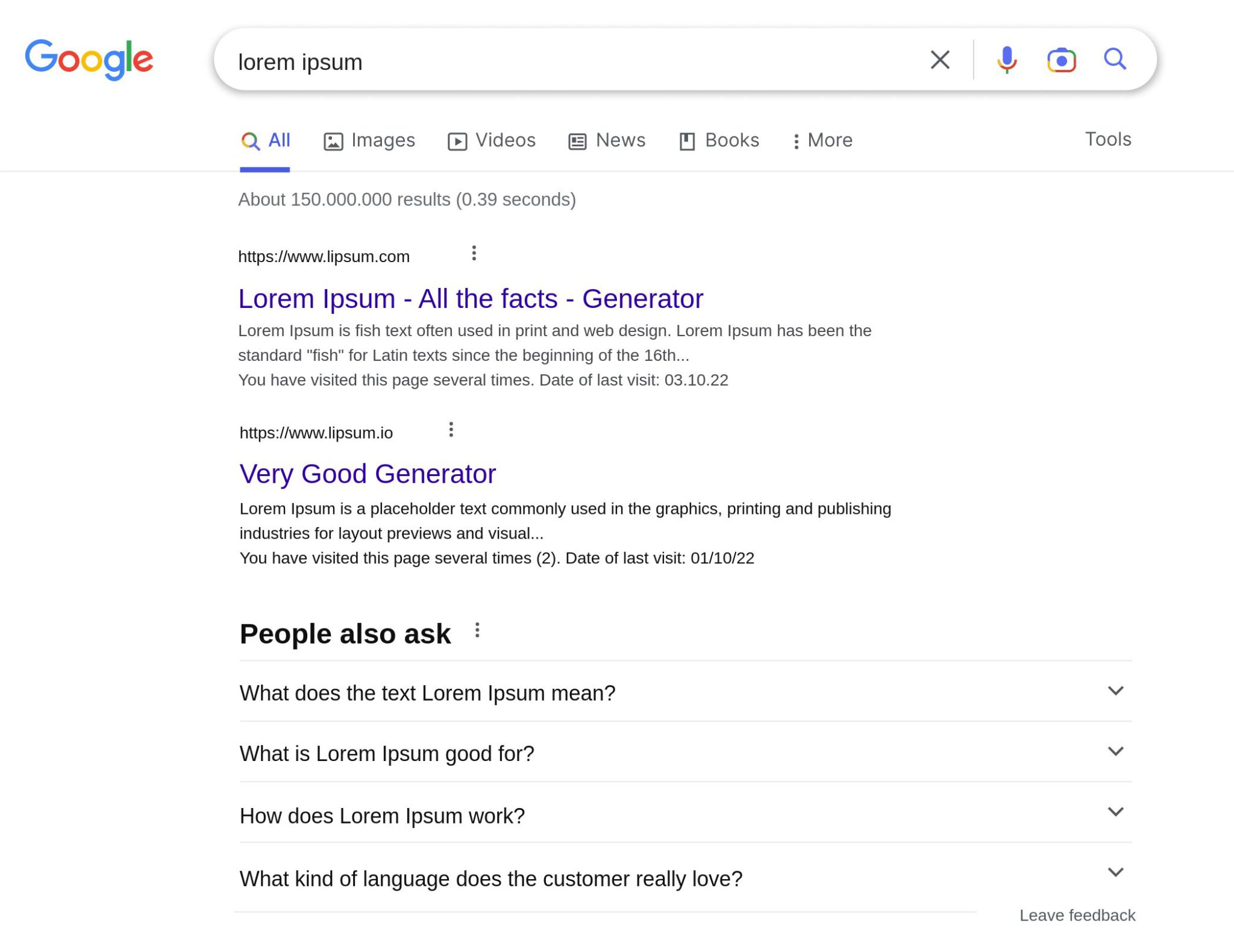The image depicts a Google search results page with the query "Lorem Ipsum" entered into the search bar. At the top, the iconic Google logo is prominently displayed next to the search bar. Beneath the search bar are navigation options for different types of search results, including All, Images, Videos, News, Books, and More.

The first search result is for the website "Lipsum.com" with the title "Lorem Ipsum - All the facts - Lipsum generator." The description explains that "Lorem Ipsum" is dummy text frequently used in print and web design, tracing its origins back to the early 16th century. It is noted that the user has visited this page several times, with the most recent visit dated March 10, 2022.

The second search result is for the website "Lipsum.io" featuring the title "Very good generator." This result highlights that "Lorem Ipsum" is placeholder text commonly utilized in the graphics, printing, and publishing industries for layout previews and visual aesthetics. The user has also visited this page multiple times, with the latest visit recorded on January 10, 2022.